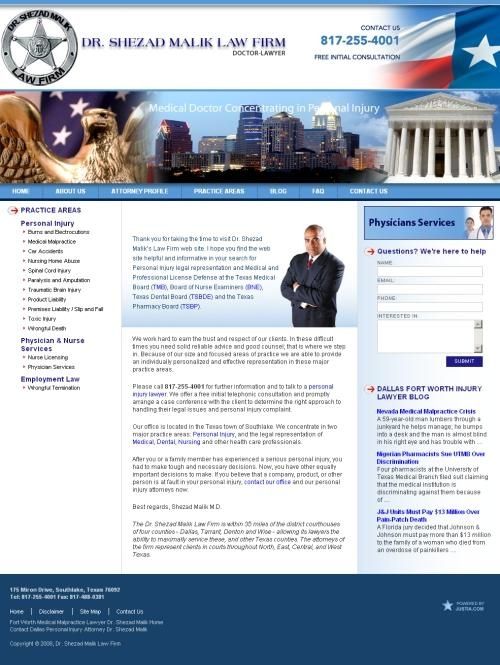Front page of the Dr. Shehzad Malik Law Firm website:

At the top of the page, a clean white banner features a Texas flag subtly blending into the background on the left. Adjacent to it, a silver sheriff's badge prominently displays "Dr. Shehzad Malik," with "Law Firm" inscribed underneath. Below, in bold blue lettering, "Dr. Shehzad Malik Law Firm" and the title "Doctor/Lawyer" are prominently shown. To the right, the contact information "Contact Us: 817-255-4001" is provided, including the offer of a free initial consultation.

A secondary banner located directly below showcases multiple images, including an eagle, a cityscape, and a governmental building, accompanied by the text "Medical Doctor Concentrating in Personal Injury."

Under this banner, a set of navigational links appears, including: 
- Home
- About Us
- Attorney Profile
- Practice Areas
- Blog
- FAQs
- Contact Us

On the left side of the page, additional links provide further details about Dr. Malik's personal injury law practice and his medical qualifications.

In the center of the page, a professional photograph of Dr. Shehzad Malik is accompanied by extensive information detailing his qualifications and services.

On the right side, the section titled "Physician Services" invites visitors to ask questions by entering their name, email, phone number, and interests. Additional links are available for more information.